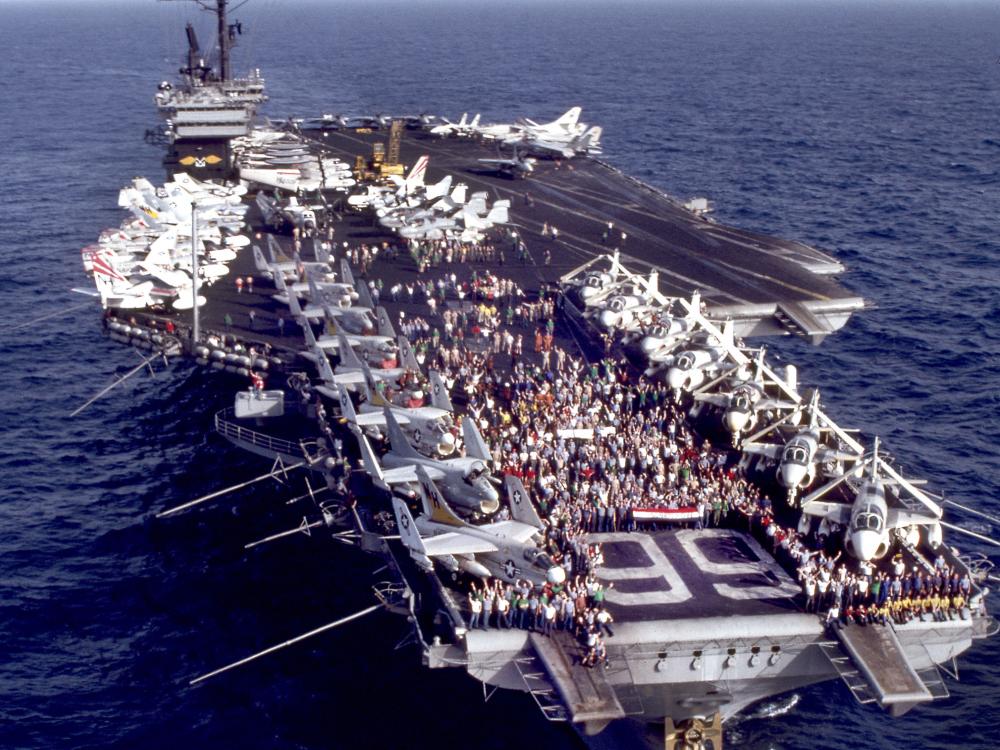This photograph captures a top, diagonal view of a massive aircraft carrier, identified by its prominent runways and sheer size, stationed in the middle of a vast, dark blue ocean with no other land or vessels in sight. The deck is lined with dozens of aircraft, including at least 20 fighter jets arranged diagonally along the ship's edge and roughly seven to eight helicopters situated on one side. A notable feature is the two large runways—one diagonal and one straight—that span the length of the deck. In the back left corner, a communications tower stands tall, overseeing the operations. At the front of the ship, the number "99" is clearly visible. The scene is bustling with activity as a large crowd of people is gathered on deck, potentially indicating a celebration or event, suggesting the carrier is host to hundreds of personnel.